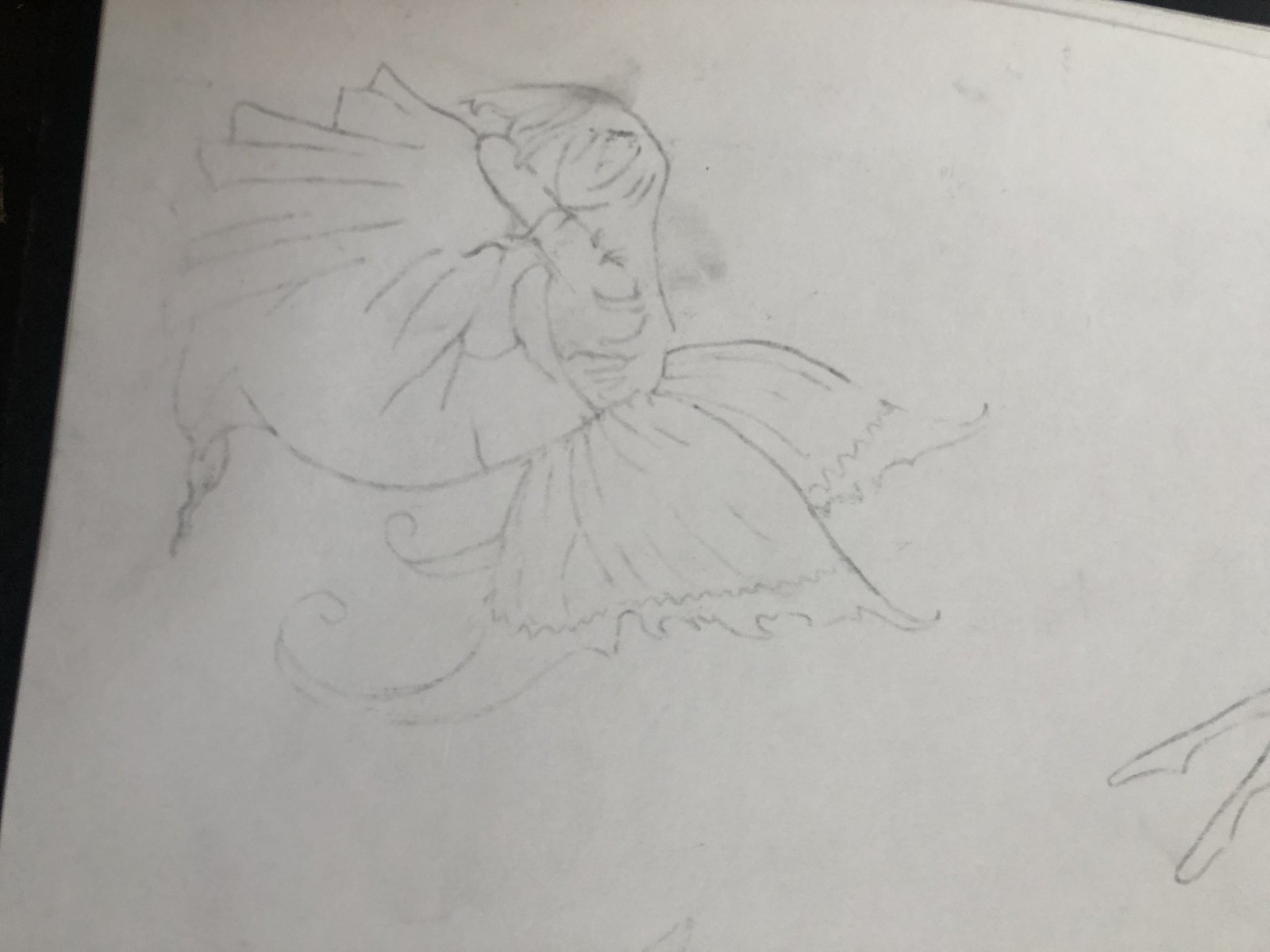A delicate pencil sketch, lightly rendered on white parchment-like paper set against a black background, captures a horizontal scene brimming with intricate details. The central figure, adorned in a long, flowing dress, is depicted in a kneeling position upon an indistinct object resembling a skirt. This figure is ethereal, bearing butterfly-like wings that add a touch of whimsy and fantasy. The head of the figure rests gently on folded arms, exuding a sense of serene repose. In the lower right corner of the composition, a pair of feet and calves subtly peeks into the scene, adding an element of intrigue and balance to the artwork.